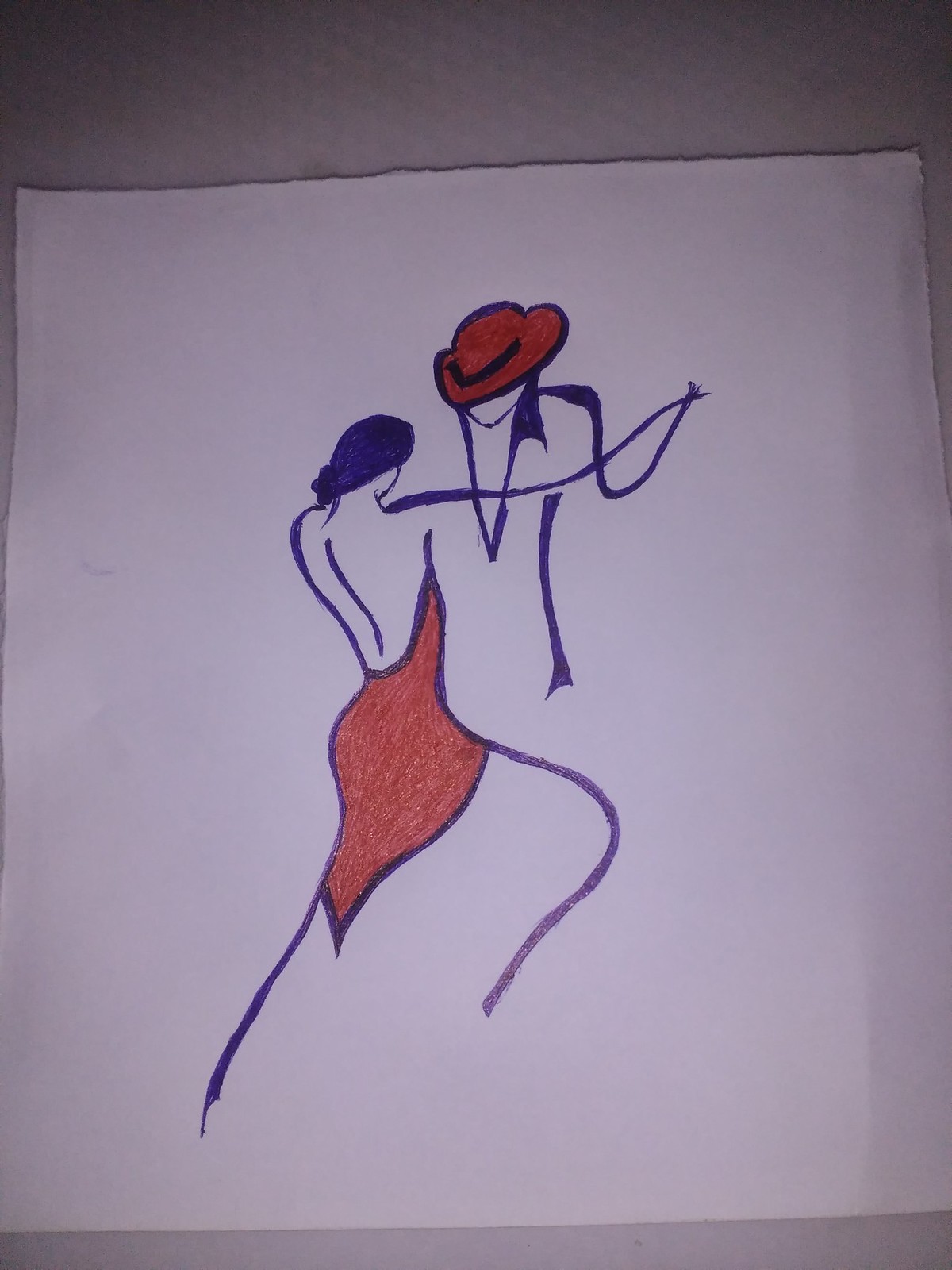This artistic illustration captures a surreal and evocative scene of a man and woman dancing. The figures are rendered in an expressive palette of red, bluish-purple, and hints of black, blending abstract and figurative elements. The man stands out with his red hat and a collared shirt featuring a deep V-neck, his minimalistic arm depicted as a squiggle. The woman is elegantly adorned in a red dress, her hair neatly tied up, with her legs abstractly represented by curved lines. The drawing, set against a white background, gives the impression of partially outlined forms in motion, creating a dynamic and captivating visual experience. The piece demonstrates a unique blend of surrealism and artistic finesse.